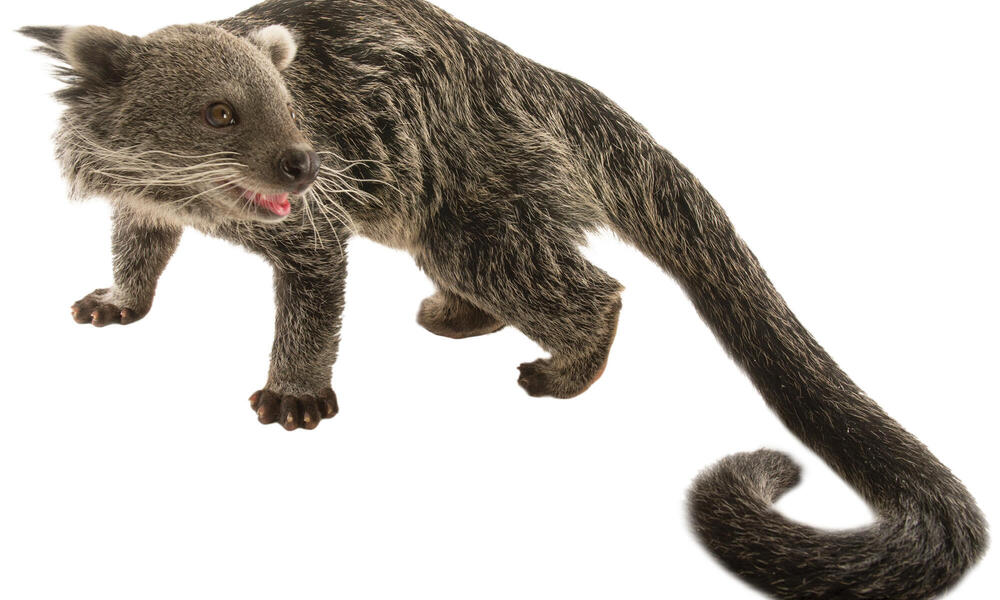The image features a gray, fierce-looking creature with an ambiguous origin, possibly either a real animal or an artistic creation. The animal stands sideways at a slight angle, its front legs set wide apart in a stance that exudes aggression and a "don't mess with me" attitude. Its head is turned over its left shoulder, revealing bared teeth and long white whiskers. The creature has bear-like ears and a muzzle resembling that of a weasel or polecat, though not exactly the same. It boasts a stripy gray coat and a remarkably long tail that curls around prominently in the foreground.